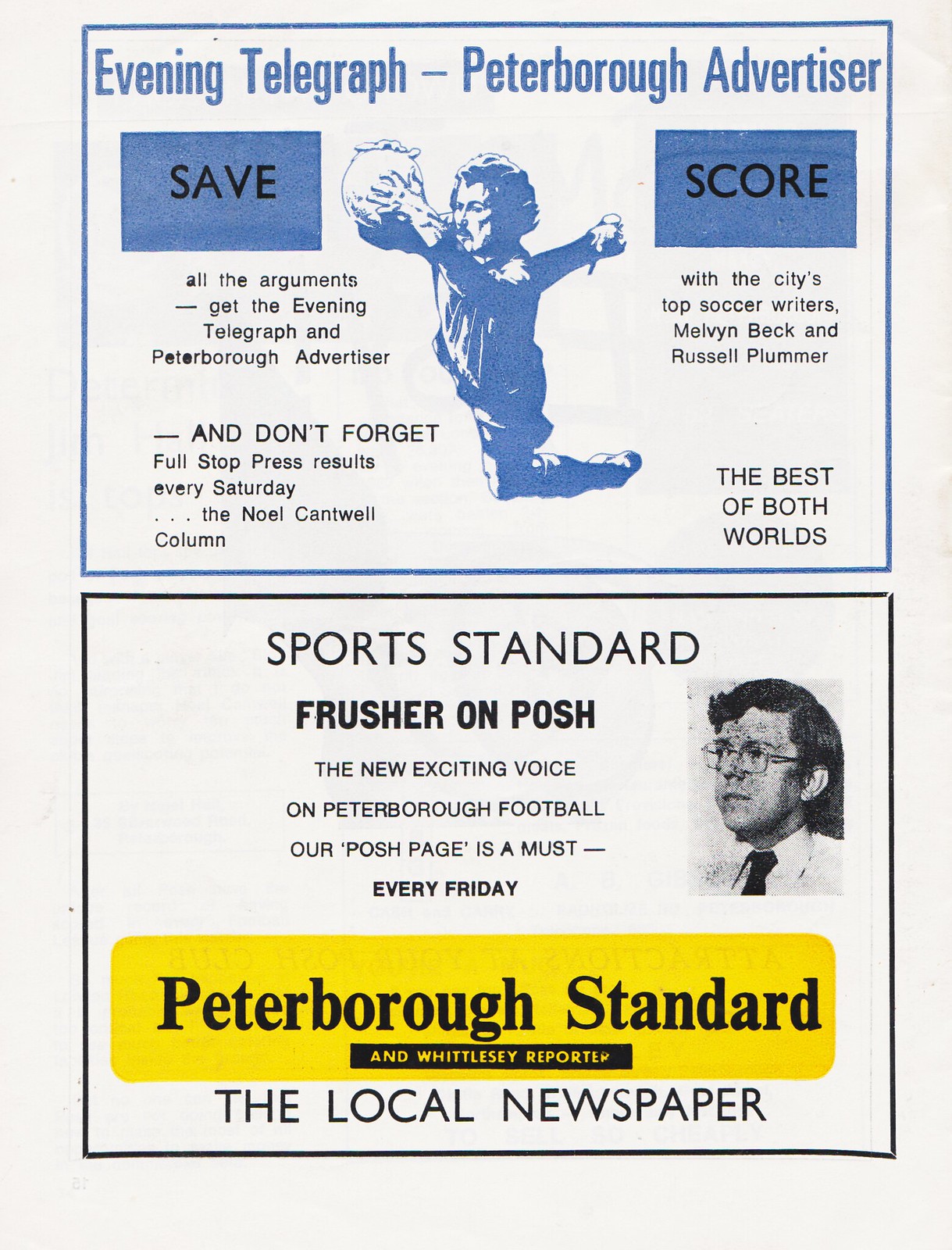This image features an old newspaper advertisement with two main sections. The top section is outlined in blue with text in both blue and black, set against an off-white background. It announces the "Evening Telegraph Peterborough Advertiser" and prominently features a small image of a person jumping to catch a ball. Captioned "Save. All the arguments—get the Evening Telegraph and Peterborough Advertiser," it highlights features such as "Full-stop press results every Saturday" and promotes columns by writers Melvin Beck and Russell Plummer, described as providing "the best of both worlds."

The bottom section is outlined in black and features mainly black text, with the title "Sports Standard" and the subtitle "Fresher on Posh," boasting about "the new, exciting voice on Peterborough football." It urges readers to catch "Our Posh page every Friday." Additionally, there is a yellow banner that reads "Peterborough Standard and Whitsley Reporter, the local newspaper," and it includes an image of a young man with glasses, looking to the left. This dual-section layout serves to promote the newspaper's comprehensive sports coverage and appeal to local football fans.